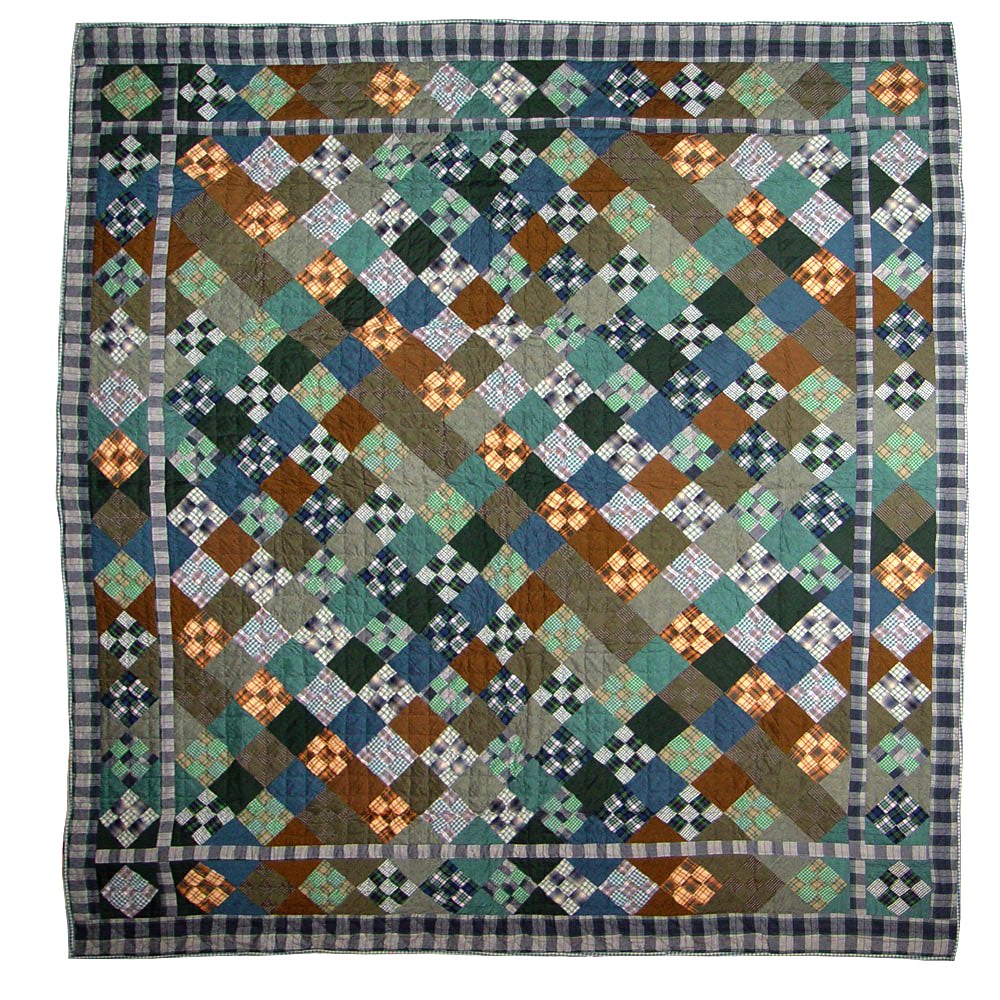The image showcases a detailed, handmade patchwork quilt, rectangular and vertically oriented. The quilt features a prominent border along its edge, approximately one to two inches wide, with blue and white stripes. Inside this is a thinner border with a similar striped pattern. The quilt's core is composed of various squares, many organized diagonally, giving a checkerboard-like appearance. These squares include a mix of solid colors and patterns, such as light and dark browns, grays, blues, and greens. Notably, some squares consist of smaller squares within them, forming intricate checkerboard and random designs. Across the quilt’s center, a diagonal row of solid squares stands out, adding a striking contrast to the overall mosaic of colors and patterns.